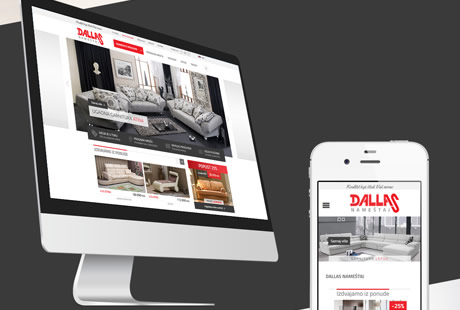On a background of dark gray, the image showcases both a desktop computer and a smartphone displaying the same website, but with different images. The desktop, resembling the design of an iMac, prominently features the word "Dallas" at the top, slightly slanted and partially obscured. Below this heading, an image of a tastefully arranged living room includes a plush sofa, a loveseat, and a chair, all adorned with numerous cushions. Underneath this main image, there are three smaller pictures: an L-shaped sofa with a high backrest, a compact two-seater leather loveseat, and a stylish chaise lounge, each displayed individually. The smartphone, also presenting the same website, highlights a distinctive U-shaped sofa, designed with two arms on either side and a middle section, serving as a central visual feature.